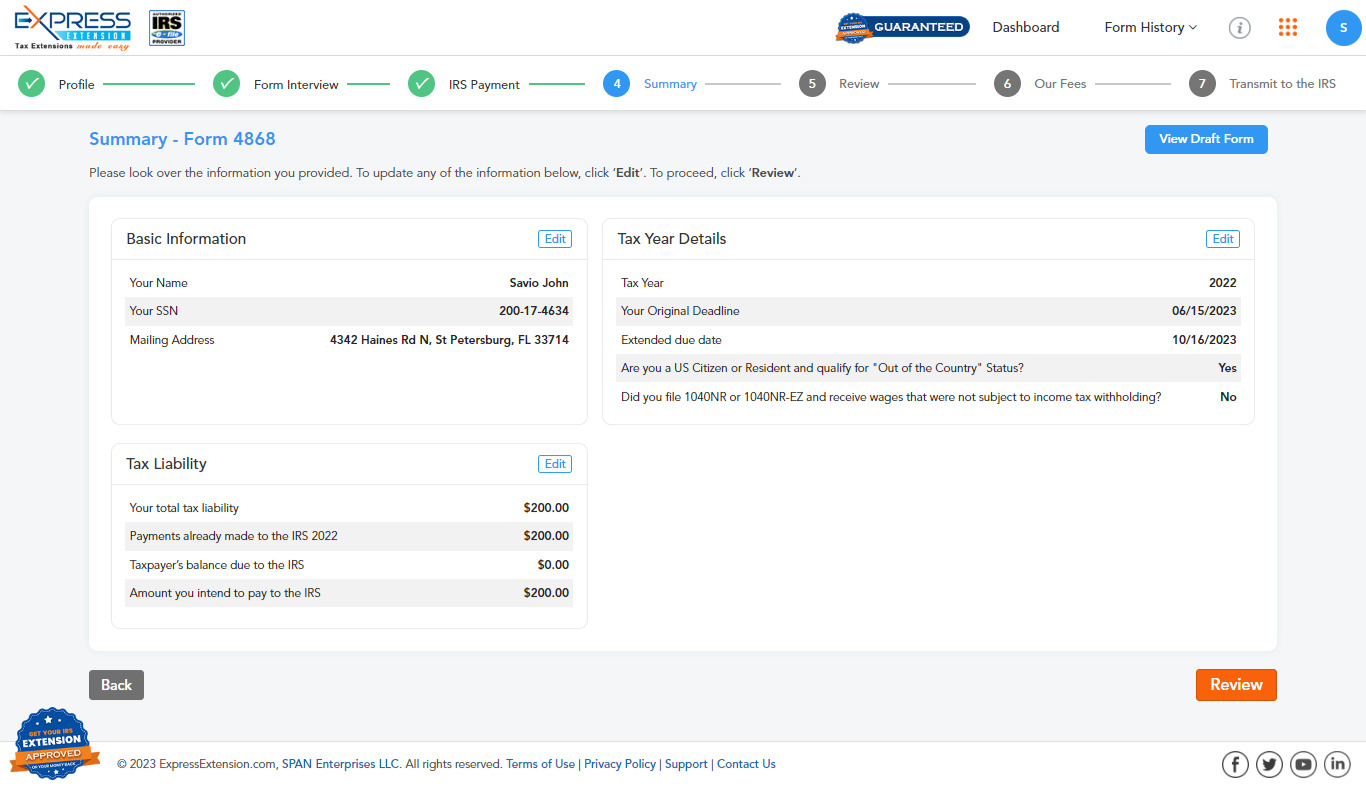Screenshot Caption:

A detailed screenshot from the website "Express Extensions," showcasing a feature for easy tax extension applications. The interface includes several sections:
 
Header: The title "Tax Extensions Made Easy" is prominently displayed.

Checklist: Three completed steps are marked with checkmarks inside circles:
1. Profile
2. Forum Interview
3. IRS Payment

Main Section: The form being reviewed is "Form 4868" under the heading "Summary." Users are instructed to review the information provided.

Basic Information: 
- Name: Savio John
- SSN: Filled in
- Mailing Address: A Florida address

Tax Liability Section:
- Total Tax Liability: $200.00
- Payments Made to IRS 2022: $200.00
- Balance Due to IRS: $0.00
- Amount Intended to Pay to IRS: $200.00

An orange "Back" button is present at the bottom of this section.

Right Sidebar: Labeled "Tax Year Details," it lists:
- Tax Year: 2022
- Original Deadline: 06-15-2023
- Extended Due Date: 10-16-2023
- Question: Are you a U.S. citizen or resident and qualify for out of the country status? Answer: Yes
- Question: Did you file 1040NR or 1040NREZ and receive wages that were not subject to income tax withholding? Answer: No

At the bottom of the sidebar, a prominent orange button labeled "Review" invites users to proceed.